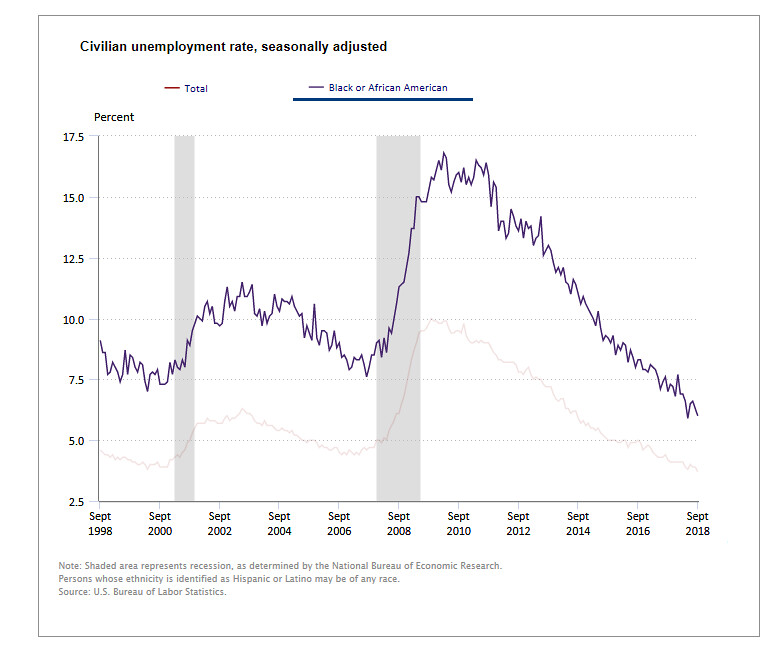This image is a detailed chart depicting the seasonally adjusted civilian unemployment rates, distinguished between total unemployment and unemployment among Black or African-American civilians, from September 1998 to September 2018. The chart, primarily in black and white, includes a few colored markers for emphasis: a small red marker labeled "total" and a small black marker, underlined in blue, labeled "Black or African-American." 

On the left side of the chart, the vertical axis starts at 2.5% and increases in intervals of 2.5% up to 17.5%. Along the bottom, from left to right, are chronological intervals starting at September 1998 and ending at September 2018. Notably, unemployment rates begin around 8-9% in 1998, experience fluctuations and see significant peaks around 2010, and then drop to their lowest in September 2018, around 6%. 

There is a shaded area on the chart representing a recession period as determined by the National Bureau of Economic Research. In small gray text at the bottom, it notes that "persons whose ethnicity is identified as Hispanic or Latino may be of any race" and that the source of the data is the U.S. Bureau of Labor Statistics. 

Overall, the chart indicates a marked spike in Black or African-American unemployment around 2010, reaching just under 17.5%, which then gradually decreased, aligning closely with the total unemployment trends by the end of the observed period. This detailed visualization underscores the variance and trends in unemployment rates over the two-decade span.